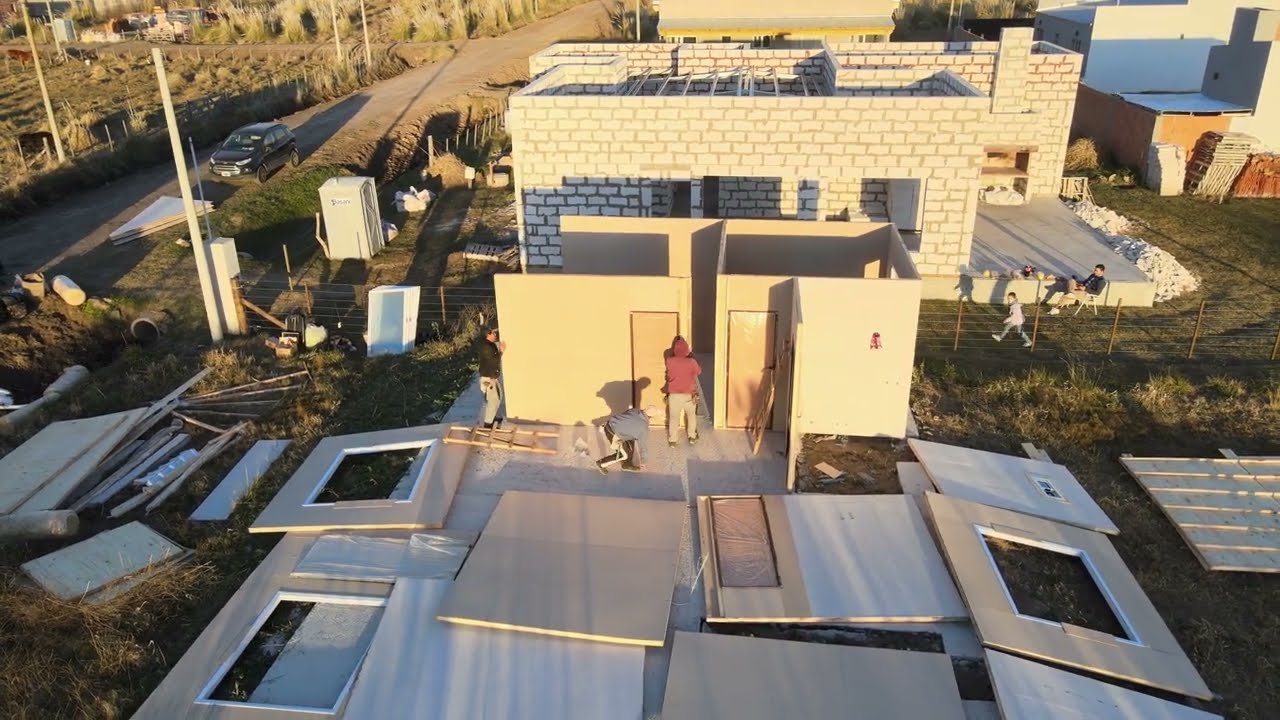In the photograph, an active construction site is captured with several individuals working on assembling what appears to be a series of small, cube-like structures that resemble rooms or closets with doors. The structures are primarily made from wooden boards and do not yet have roofs, giving them an unfinished appearance. Three men are clearly visible, each engaged in various tasks such as holding up and securing walls. The surrounding area is strewn with additional wooden pieces and squares, suggesting more structures are yet to be assembled.

In the background, there is a mix of activity: a person is seated, another person stands near a short fence, and a child walks behind it. A vehicle is seen on a road to the left, flanked by a large dirt field and bushes. Across the road lies another field with tall, bushy trees and what appears to be a commercial area or additional buildings. Behind the primary construction site, there is a grayish-white stone structure that adds to the scene's complexity.

The weather appears sunny, casting shadows across the site and highlighting the atypically thick, white brick material of the existing structures. The overall atmosphere is bustling and somewhat chaotic, with the combination of unfinished wood and unconventional block-like materials lending a slightly surreal quality to the work in progress.